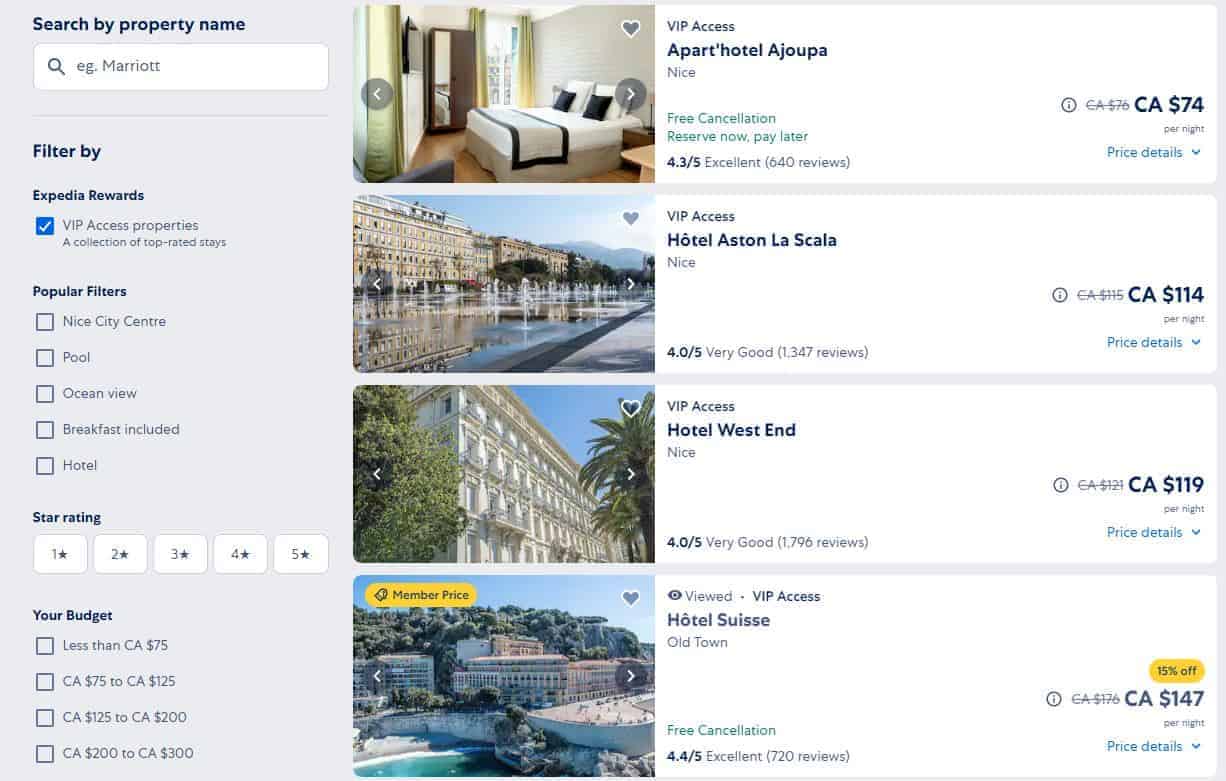The image showcases a well-organized hotel booking webpage. On the left side, there is a user-friendly search section that allows users to find hotels by property name, with an example provided (Marriott). Below the search bar is a detailed filter panel. This panel includes options to filter properties by Expedia Rewards, marked with a check for VIP access properties known for being top-rated stays. 

Additionally, there are popular filter categories like "City Center," "Pool," "Ocean View," "Breakfast Included," and "Hotel," allowing users to refine their search based on their preferences. The star rating filter enables users to select hotels ranging from 1 to 5 stars. Budget filters are divided into categories: less than CA $75, CA $75 to CA $125, CA $125 to CA $200, and CA $200 to CA $300.

On the right side, the page displays various hotel options. Highlighted properties include Park Hotel Aljopa listed at CA $74 per night with a 4.35-star rating, Hotel Aston La Scala at CA $114 per night with a 4-star rating, Hotel Westin at CA $119 per night also with a 4-star rating, and Hotel Suisse, distinguished as the highest-rated option with a 4.4-star rating at CA $147 per night. The hotels are set against beautiful Mediterranean backdrops, enhancing their appeal.